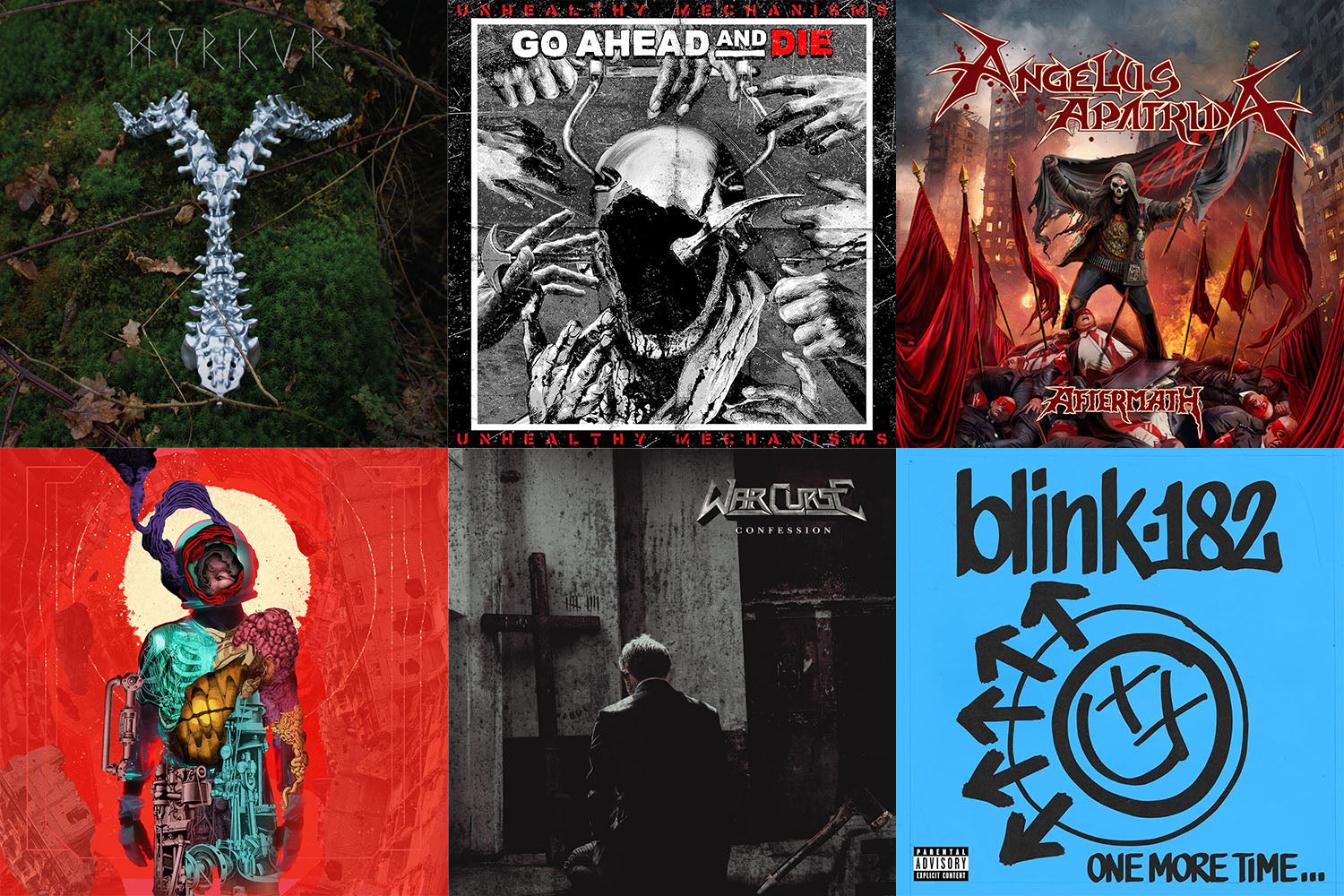This horizontal rectangular image showcases six distinct album covers arranged in a grid pattern, with three covers on the top row and three on the bottom. Each cover represents varying artistic styles and themes. 

In the upper left corner, the album "Merkur" features a metallic zipper design set against a backdrop of grass and leaves, giving it a textured and organic feel. Moving to the center of the top row, there is a black and white image titled "Unhealthy Mechanisms," depicting hands reaching out towards a hooded figure, conveying a sense of urgency and desolation. To its right, the cover for the band Angelus Apatrida presents a chaotic scene with a skull-faced figure leading a charge in a cityscape ravaged by chaos and destruction, appropriately titled "Aftermath."

On the bottom row, starting from the left, a vivid red album cover with a multicolored human form stands out, although further details about it are not clear. The center features the "War Curse: Confession" cover, showing a man in a suit staring at a cross in a stark room. Finally, the lower right corner displays the cover for Blink-182’s "One More Time," set against a blue background. This cover includes the band’s name, their iconic smiley face logo with X's for eyes, and black arrows pointing in various directions, encapsulating a sense of nostalgic anticipation and reflection.

These album covers together provide a diverse visual and thematic tapestry, highlighting the varied artistic expressions of different bands.